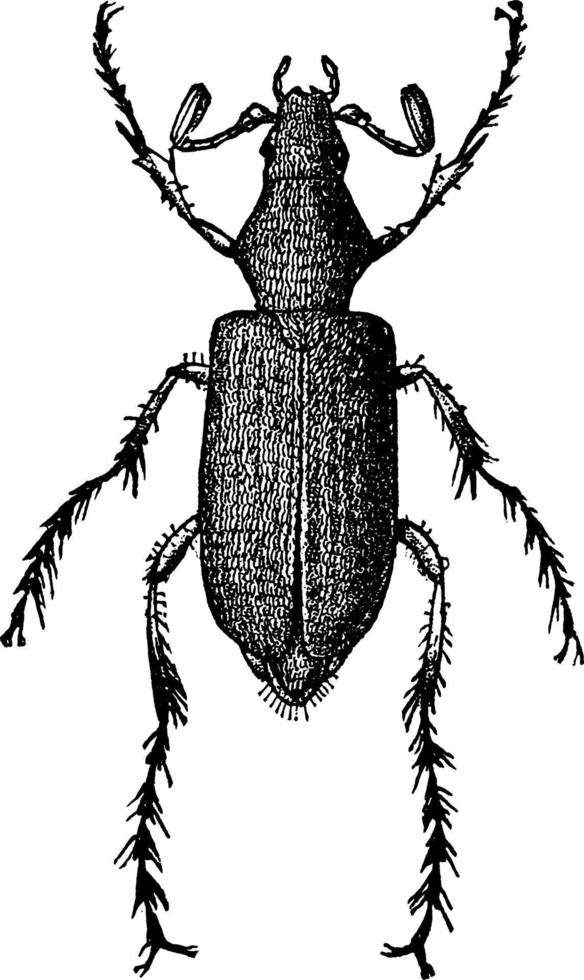This black and white sketch depicts a beetle set against a plain white background. The beetle's body is characterized by a small, semi-triangular head, which transitions into a larger, more prominent, squarish body tapering into a curved lower section. Emerging from its head are two prominent antennae, or possibly eyes on stalks, accompanied by mandibles near its mouth. Each side of the beetle features three legs adorned with hair-like structures, with the front legs appearing shorter and slightly different in shape, reminiscent of small boxing gloves. The drawing highlights the wiry, spiked details on the legs and the body's intricate textures, capturing the beetle's anatomical features despite the illustration's overall simplicity.